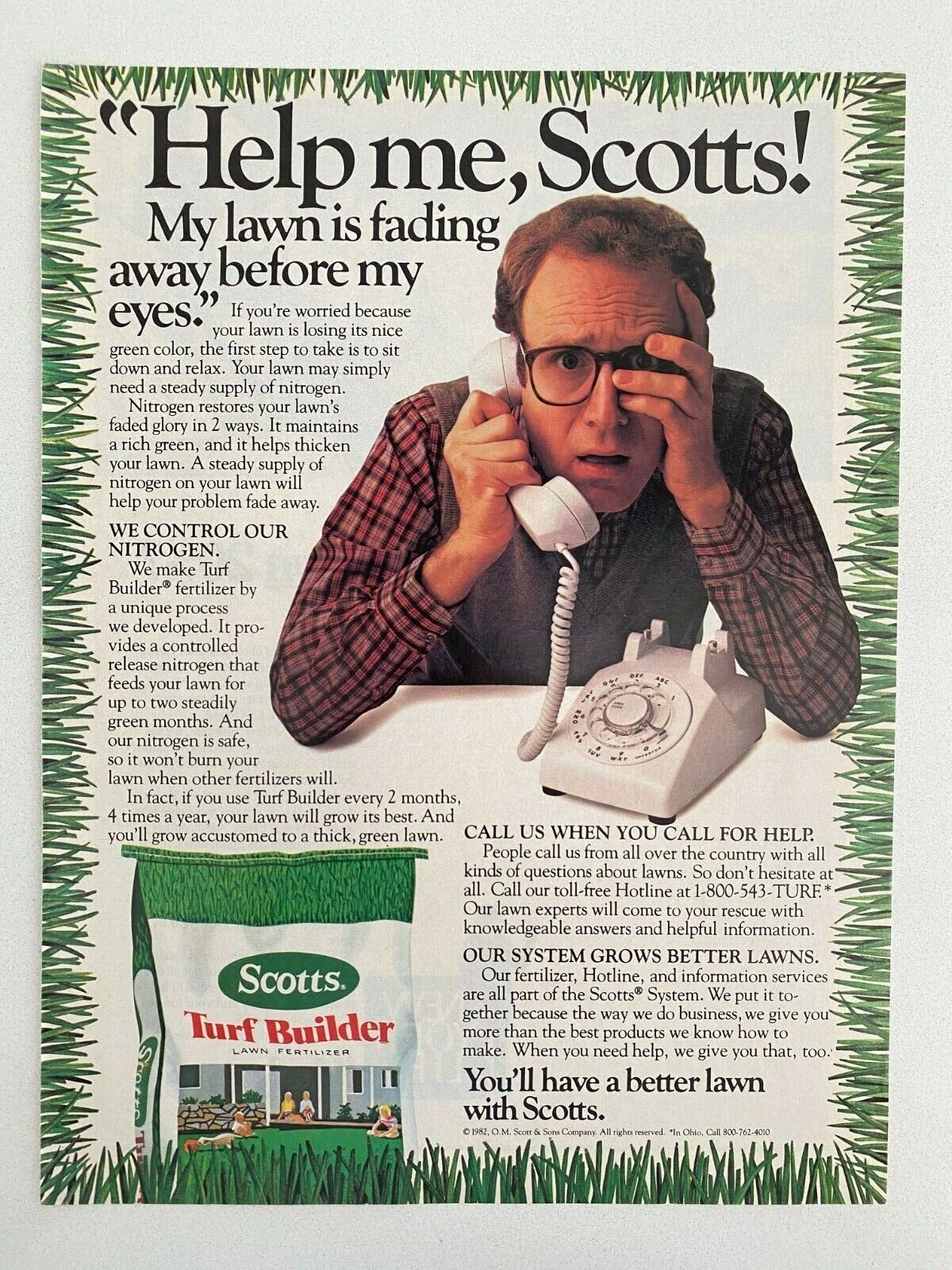This vintage advertisement for Scott's Turf Builder lawn fertilizer features a distressed man, reminiscent of Woody Allen, frantically calling for help on an old rotary phone. The man, wearing black-framed glasses, a plaid shirt, and a brown vest, leans on a counter with his left hand pressed against his head. The top of the ad reads, "Help me Scott, my lawn is fading away before my eyes," in bold black letters. The border of the ad is made up of individual blades of green grass, creating a lush, nature-inspired frame around the white page. In the bottom left corner, there's a green and white Scott's Turf Builder bag, showing a vibrant front lawn with children and a family enjoying the outdoors. The tagline at the bottom right promises, "You'll have a better lawn with Scott's."